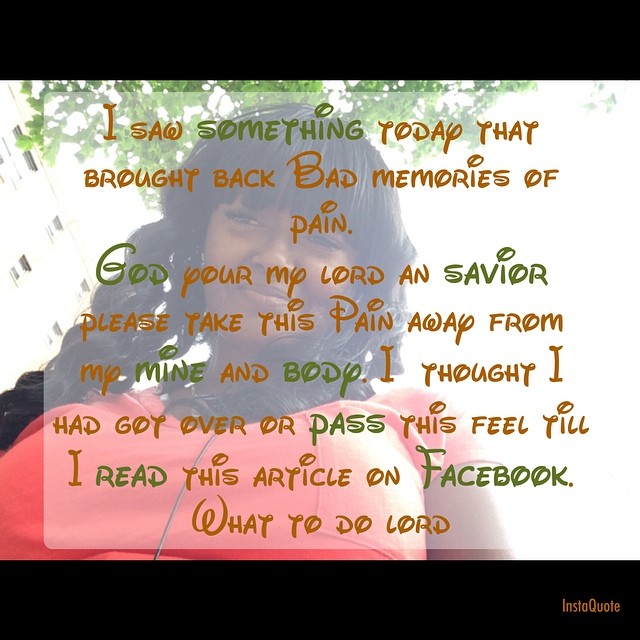The image is a social media graphic featuring a young African American woman in a pink top with a zipper, set against an outdoor backdrop with trees. Encasing the image are solid black borders at the top and bottom, with "InstaQuote" written in the bottom right corner. The central focus is on the woman looking towards the camera. Overlaying her image is a poignant message in a Walt Disney-style font with large circular dots above the "i's," rendered in orange and green text. The message reads: "I saw something today that brought back bad memories of pain. God, poor my Lord and Savior, please take this pain away from my mind and body. I thought I had got over or past this feel till I read this article on Facebook, what to do Lord." The graphic, likely created in a program like PowerPoint, is intended as a heartfelt social media post and is clearly designed to be shared widely.